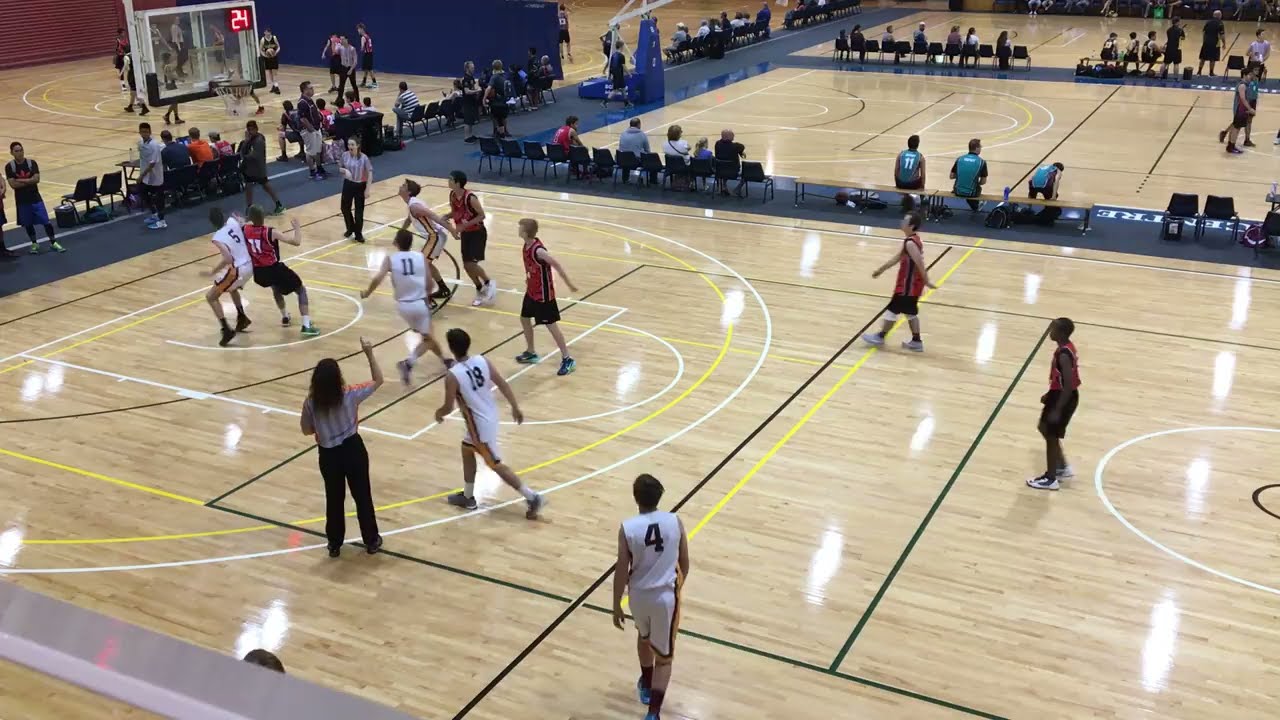The photograph captures a high-energy, multi-game basketball scene from an elevated vantage point, likely from the bleachers. The main court in the forefront, lit by bright overhead lighting reflecting off the shiny beige wooden floor, features a heated match between a white team with black numbers (players 5, 11, 18, and 4) and a red team with white numbers and black stripes (though their numbers are obscured). A scoreboard shows "24" in a red square with white numerals. One referee has their hand raised while the other stands under the basket. The ball appears to be lodged in the net, and the referee seems to be making a call. Surrounding this main action, there are four additional courts, each separated by rows of chairs and benches, with more games in progress. Spectators can be seen seated on both sides of these courts, creating a bustling and dynamic atmosphere typical of middle or high school tournaments.